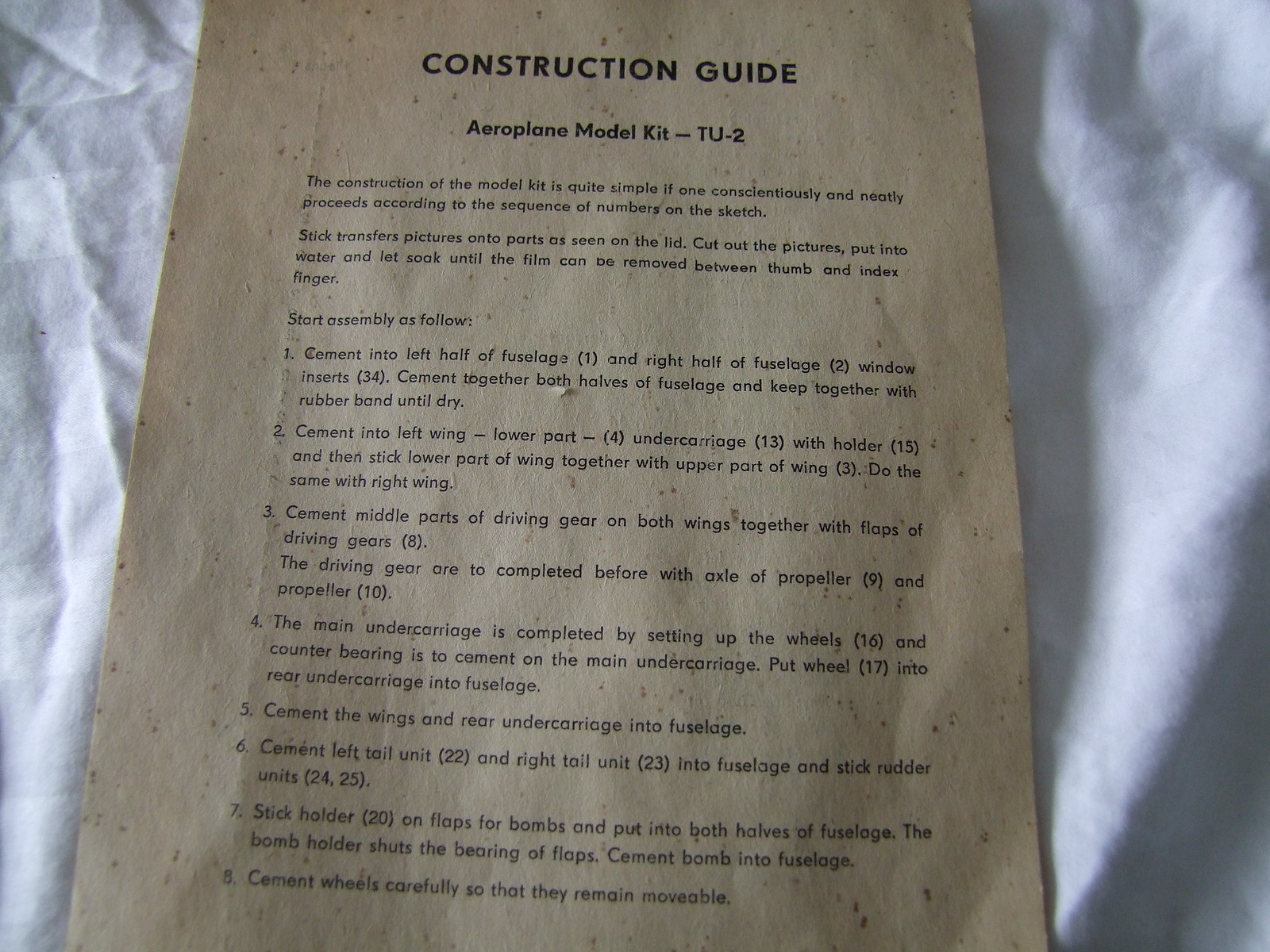The image depicts an old, slightly wrinkled piece of paper laid on a similarly wrinkled tissue paper background. At the top of the page, in large, bold black capital letters, the title reads "CONSTRUCTION GUIDE." Just below, in smaller yet bold letters, it states "Airplane Model Kit-TU-2."

Proceeding down the page, there is a detailed set of instructions for assembling the model kit, beginning with a note that emphasizes the simplicity of the construction process when following the numbered sequence on the sketch. The introductory paragraph advises to "stick transfer pictures onto parts as seen on the lid, cut out the pictures, put into water, and let soak until the film can be removed between the thumb and index finger."

Following this, the page lists step-by-step assembly instructions, numbered from 1 to 8:

1. Cement the left half of the fuselage (part 1) and the right half (part 2), adding window inserts (part 34). Cement both halves together and secure with a rubber band until dry.
2. Cement the lower part of the left wing (part 4) and the undercarriage (part 13) with holder (part 15). Attach the lower and upper parts of the wing (part 3). Repeat this step for the right wing.
3. Assemble the middle parts of the driving gear on both wings, including the flaps (part 8), the axles of the propellers, and the propellers themselves (parts 9 and 10).
4. Complete the main undercarriage by setting up the wheels (part 16) and cementing the counter bearing. Insert the rear undercarriage wheel (part 17) into the fuselage.
5. Cement the wings and rear undercarriage into the fuselage.
6. Attach the left and right tail units (parts 22 and 23) to the fuselage and stick the rubber units (parts 24 and 25).
7. Attach the bomb holder (part 20) to the flaps and insert them into the fuselage. Cement the bomb into the fuselage.
8. Cement the wheels carefully to ensure they remain movable.